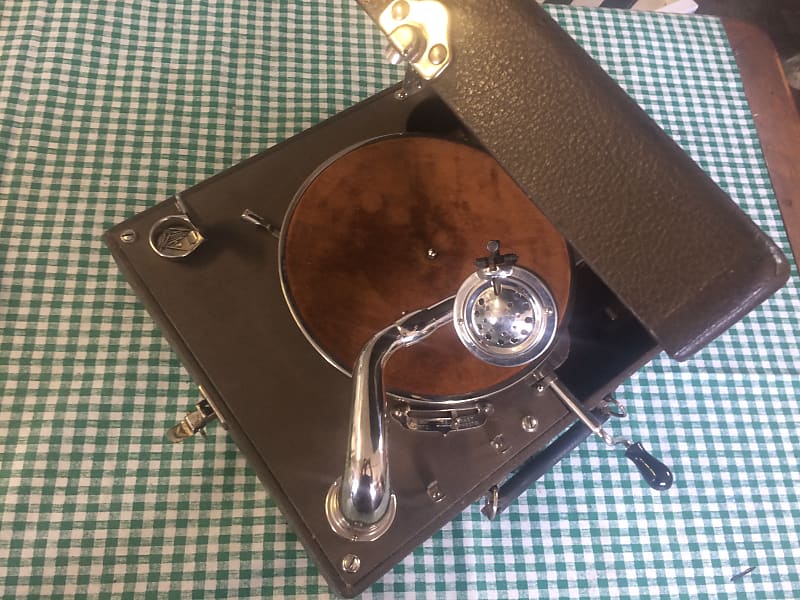The image depicts an old phonograph housed in a brown leather box with a lid that can be clamped shut. The box features a small, silver-plated record handle that might actually be made of real silver. This handle is complemented by another metal crank which sticks out of the box and is hand-cranked, a sign of the phonograph's antiquity. The handle itself is black with silver rings. Additionally, there's a small cup on one corner of the box that opens and closes, likely for storage purposes. The contraption, including the dark needle or stylus positioned in a silver tray, sits atop a green and white checkered tablecloth on a rich, dark brown wooden table. The player’s internal tray has a distinct brown, circular area, adding to the vintage aesthetic of this meticulously detailed phonograph.